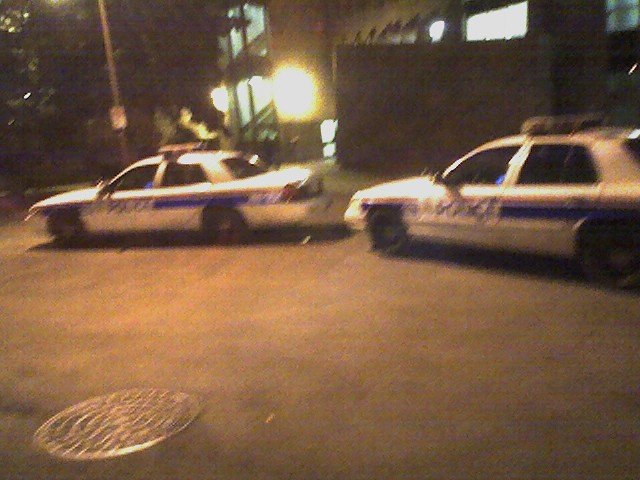This is a color photograph taken at nighttime outdoors, capturing a street scene in front of an apartment complex. The primary focus is on two white police cars positioned one behind the other, centered in the image. Both cars have a traditional police design, with blue stripes along their sides and light bars on top, but their lights and sirens are turned off. The scene is slightly out-of-focus, lending a vintage feel to the photo and making finer details such as potential text unreadable.

At the bottom left of the image, there is a manhole cover embedded in the street's blacktop or concrete surface. On the upper left corner of the photograph, a large tree and a street pole can be observed. Despite the nighttime setting, the area is dimly lit by a high-pressure sodium streetlight, casting a characteristic yellow-orange glow and creating pronounced shadows. The apartment building in the background has illuminated windows, indicating occupancy. No people are visible inside the cars or in the surroundings, making the scene appear still and quiet.